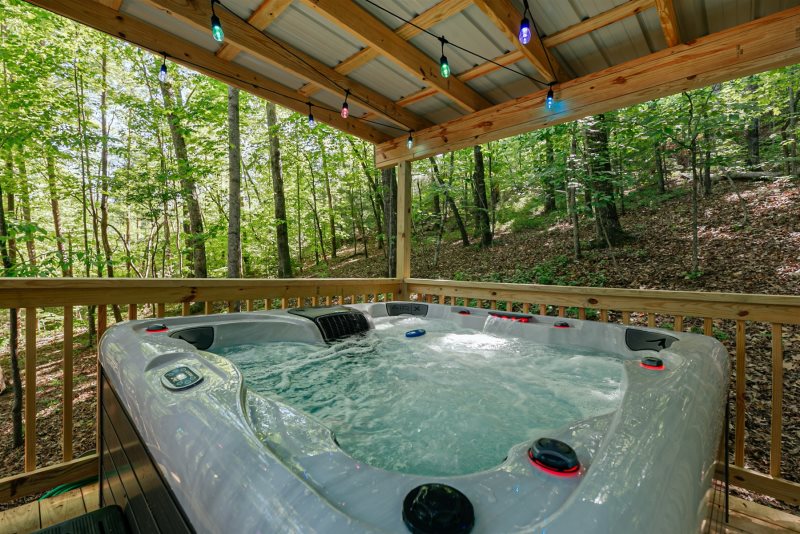This image features a large white hot tub situated in a natural, wooded area, possibly on a slope in a mountainous region. The hot tub is accompanied by rippling water and several drink holders along its edge. A settings pad is located on the left side. Surrounding the hot tub is a wooden deck and a wooden roof structure, framed by wooden beams and a metallic material on top, providing partial protection from the elements. Though the sides are open, allowing wind and rain to potentially enter, the roof offers some shelter. Adding a touch of whimsy, colorful string lights in shades of blue, purple, green, and pink are strung beneath the roof, creating a cozy and inviting ambiance, especially in the evening.